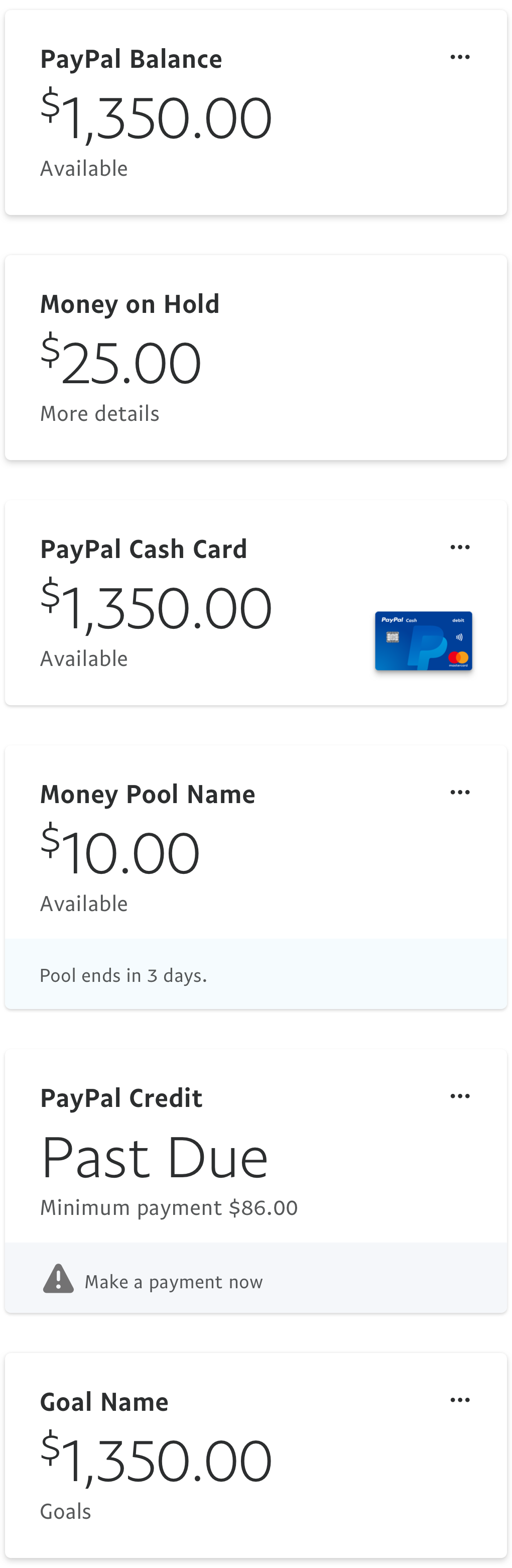The image displays a section of a financial management website, featuring various balances and financial tools, each enclosed in separate white boxes outlined in gray. 

1. **PayPal Balance**:
   - **Available**: $13.50
   - **Additional Detail**: Below, there is a box showing "Money on hold" with an amount of $25. There's also a clickable link for "More details".
   
2. **PayPal Cash Card**:
   - **Available**: $13.50
   - **Visual**: An image of a blue credit card with a small orange segment is present here.
   
3. **Money Pool**:
   - **Name**: Not specified
   - **Available**: $10
   - **Additional Info**: A blue bar at the bottom indicates that the pool ends in three days.
   
4. **PayPal Credit**:
   - **Status**: Past due
   - **Minimum Payment**: $86
   - **Call to Action**: A "Make a payment now" prompt, with an alert symbol (a triangle with an exclamation point), indicates urgency.
   
5. **Goal Name**:
   - **Available**: $13.50
   - **Note**: The term "Goals" is indicated below the balance.

Each box, except the one for the PayPal Cash Card, has a trio of dots in the top right corner for further interactions or additional options. The purpose behind listing these balances in a linear fashion and their relevance is not immediately clear from the image.